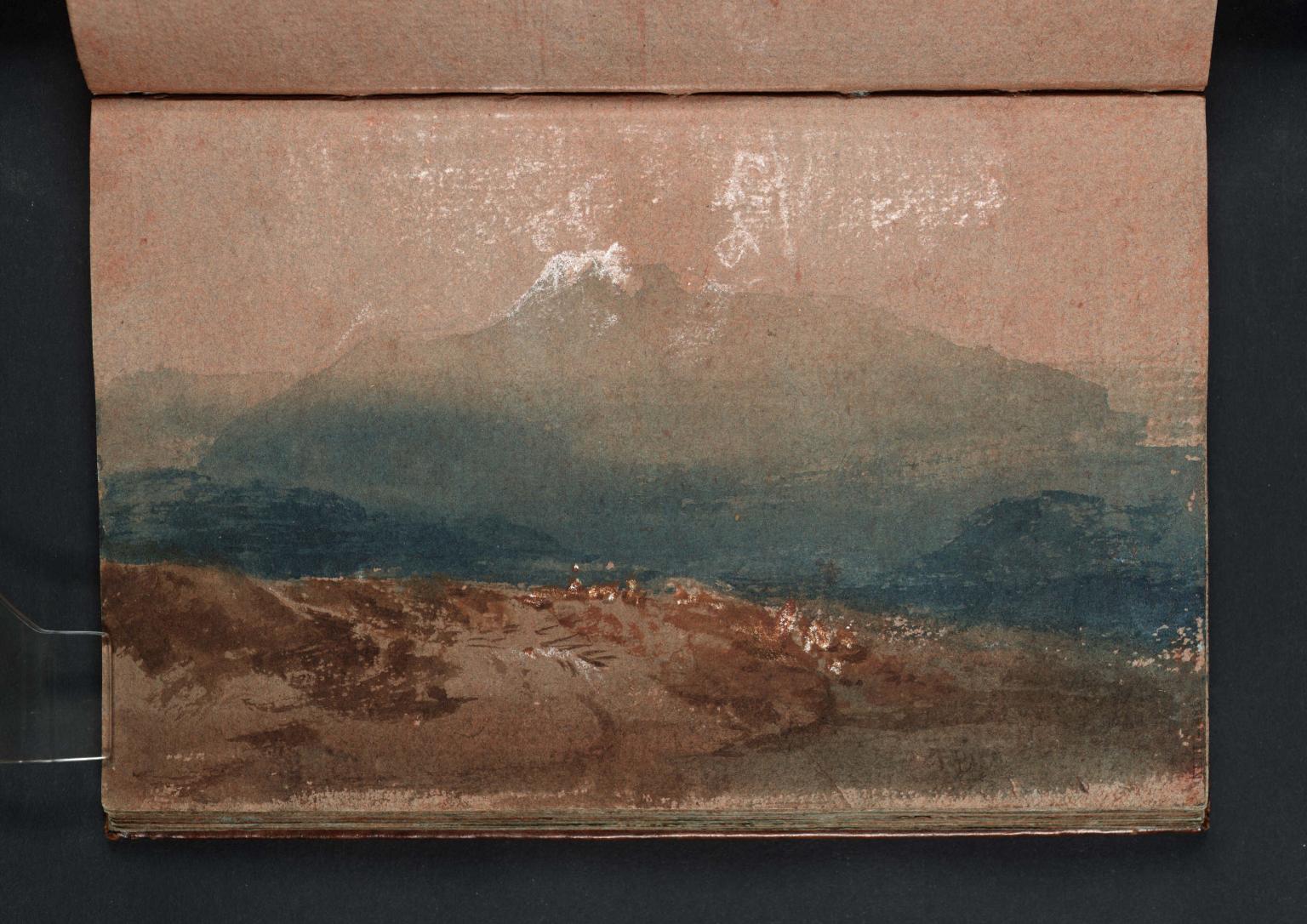The image showcases a painting nestled within an art sketchbook, notable for its vivid colors and layered composition. The sketchbook's page is largely a pinkish-reddish hue, partially obscured by a glare from a light source above. This painted page occupies the foreground, displaying a rich brown terrain that appears to be a hill or dirt trail extending across its bottom half. The earthy tones evolve into varying shades of blue as the landscape transitions into a mountainous region. These blues start dark and gradually lighten, suggesting depth and distance, culminating in a blurred, reddish sky. A partial glimpse of another page or the cover of the notebook is visible at the top of the image. The entire scene captures a blend of colors and textures, from the earthy browns to the faintly painted grey-blues, creating an intricate and dynamic visual experience.